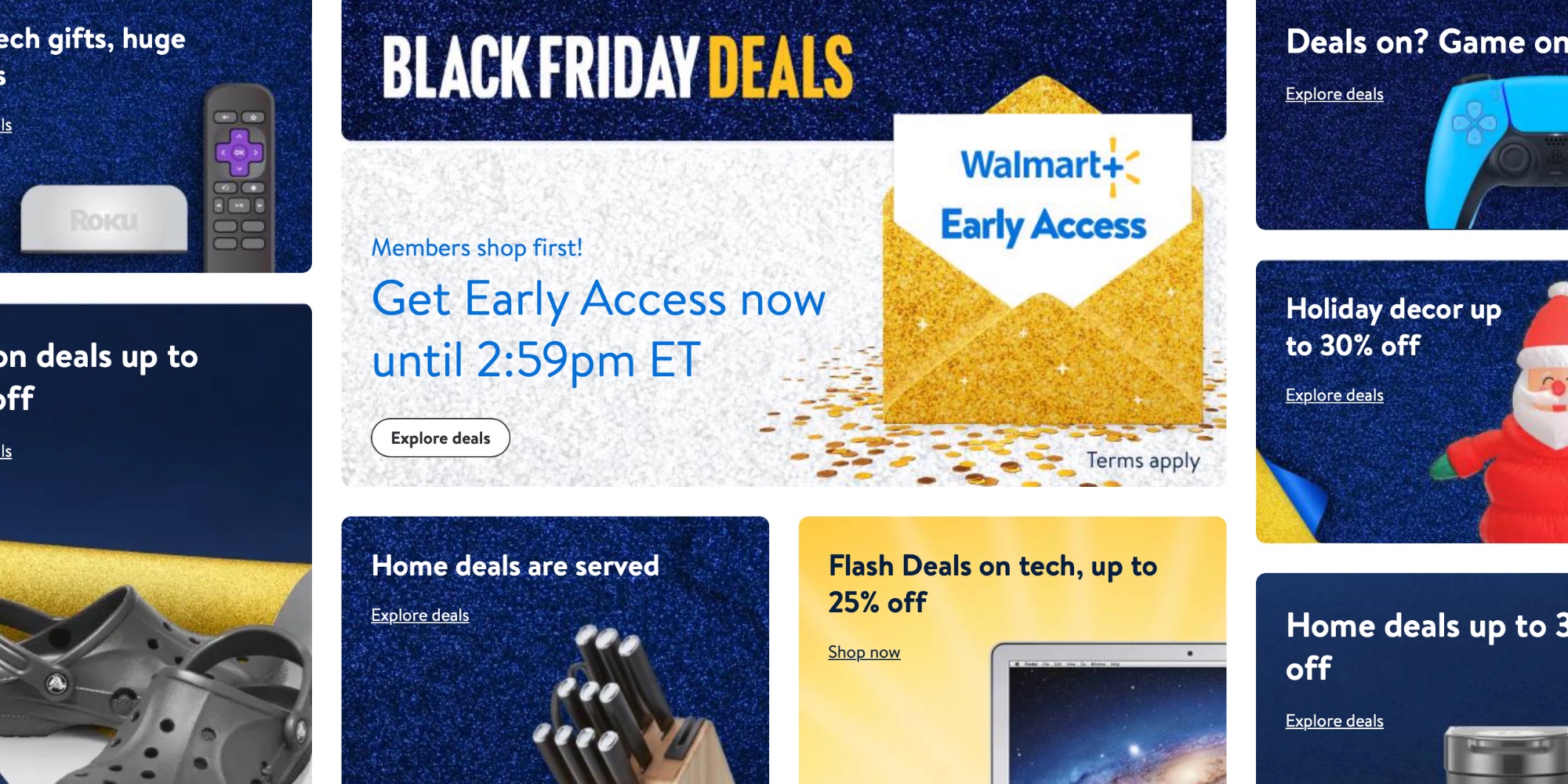The image captures a promotional display for Walmart's Black Friday deals. Centered in the photo is a large gray box with the text "Members Shop First - Get Early Access Now Until 2:59 PM Eastern Time." Below this message is a small "Explore Deals" button. To the right of this central box, there is an illustrated opened gold envelope with a letter emerging from it, labeled "Walmart Early Access."

Above the central gray box is a blue square that announces "Black Friday Deals." Surrounding the central box are various smaller boxes featuring different deals, each in distinct colors. Most of these boxes are blue; one prominently states "Home Deals." Another square, the only yellow one, reads "Flash Deals on Tech - Up to 25% off." Additionally, there are boxes advertising "Deals on Games" and "Holiday Decor - Up to 30% off."

The photo provides a vivid array of color-coded deals, highlighting the special early access Walmart members receive for Black Friday shopping.